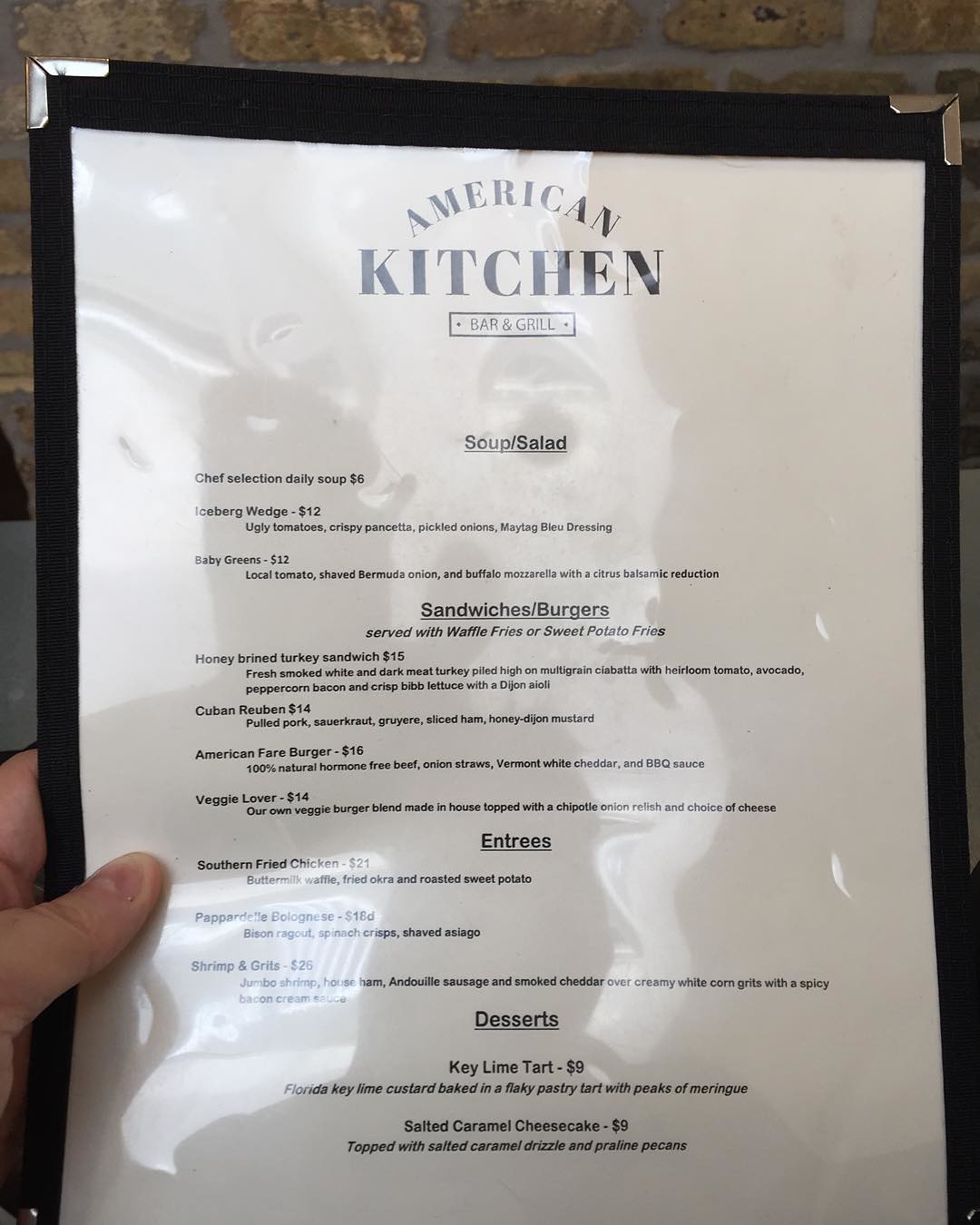A laminated menu encased in a plastic cover, secured by clip holders at the top corners, is prominently featured in this image. The menu belongs to "American Kitchen Bar and Grill" and starts by presenting the soup and salad selections, which include options like Chef Salad, Iceberg Wedge, and Baby Greens. The menu is shown with a human hand holding it, thumb in front and fingers at the back. Light reflections are visible due to a slight dent where the hand grasps the menu, particularly illuminating the sections displaying sandwiches and burgers, such as a Reuben, the American Fair Burger, and a turkey hoagie. The bottom of the menu lists desserts, featuring a Florida Key Lime Custard Tart baked in a flaky pastry and a Salted Caramel Cheesecake. Despite the small font, the text remains legible, providing a clear and detailed look at the offerings.